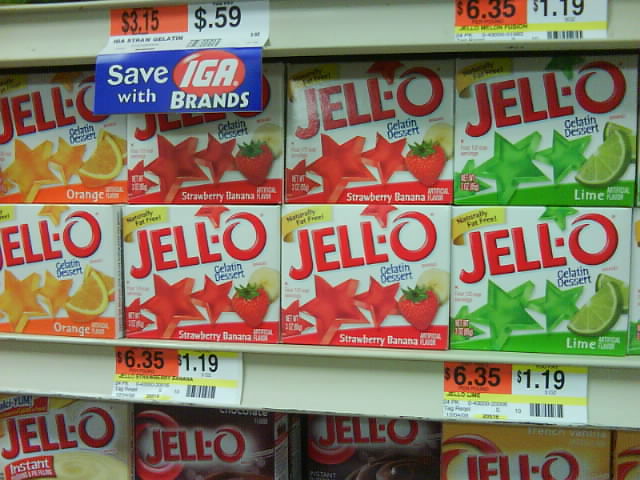This image features a section of shelving at an IGA grocery store dedicated to Jell-O products. The compact shelf only accommodates two small square Jell-O boxes in height before the next shelf starts. Prominent signage above the products reads "Save with IGA Brand," indicating a potential store promotion. Jell-O is priced at $1.19 per box, equating to $6.35 per unit.

The shelf prominently displays three flavors of Jell-O: orange, strawberry, and lime. A total of eight Jell-O boxes are arranged in the middle section: two are orange, four are strawberry, and two are lime. Additionally, there are boxes of Jell-O pudding in various flavors, including French vanilla, chocolate, and tapioca, adding variety to the selection.

The overall display is neatly organized, showcasing a colorful assortment of Jell-O options against the backdrop of the store's promotional signage.